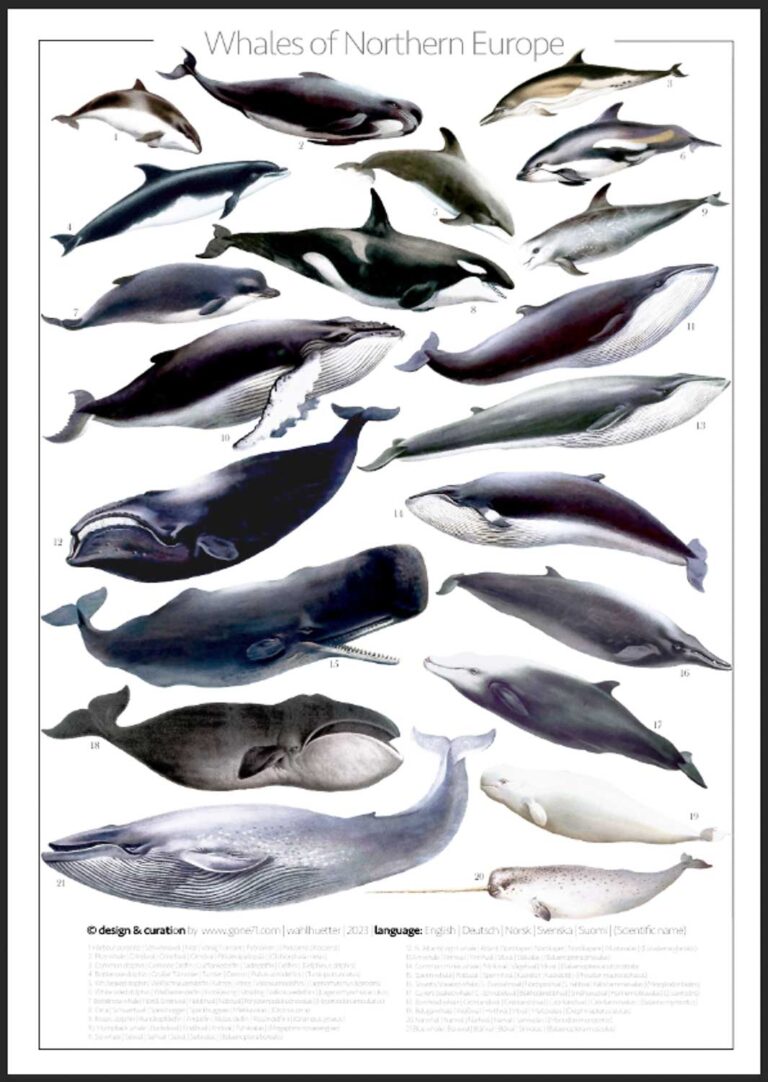The image is a portrait-oriented poster with a narrow black frame and a white background. At the top, bold black text reads "Whales of Northern Europe." The poster features detailed drawings of approximately 21 different whales, depicted in various shades of black, white, and blue. The whales are arranged primarily in two columns, though some rows contain three whales. Each whale is uniquely depicted, with varying sizes, mouth positions (some open, some closed), and tail orientations (straight or curved). At the bottom of the poster, there is a block of small, hard-to-read black text, likely providing descriptions and labels corresponding to each numbered whale illustration. The drawing style and layout provide an informative and visually engaging guide to the diverse whale species found in northern European waters.